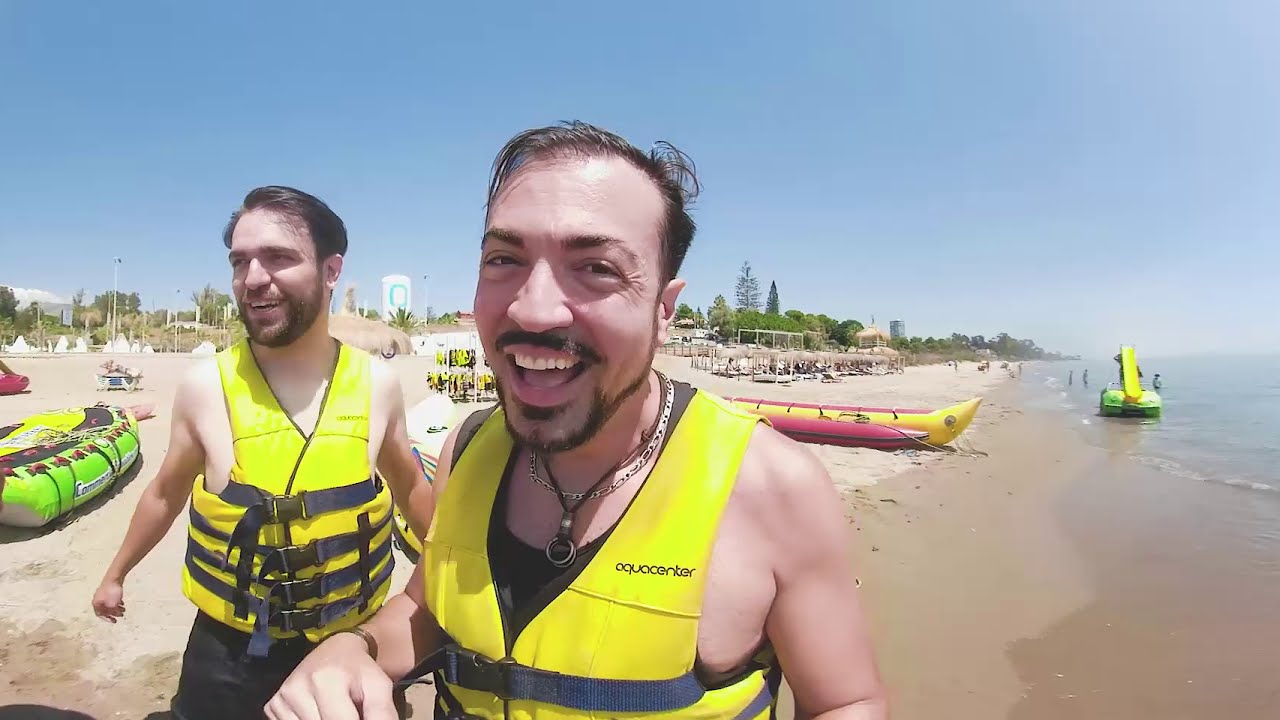In this vibrant beach scene, we have an image of two men, both with short brown hair and beards, standing on the sandy shore under a clear, blue sky. They are enjoying a sunny day at the beach, each wearing yellow life vests marked with "Aquacenter" in black, and black shorts. The man in the foreground is grinning directly at the camera, showcasing a gold necklace and a black or leather strap necklace with rings attached, as well as a bracelet, while his companion stands behind him, looking to his right and smiling. Surrounding them is a bustling beach environment with various inflatable boats, including a yellow and red raft and a red canoe. There's also a visible green and yellow raft, and in the distance, numerous palm trees and buildings can be seen. The sandy beach, dotted with people enjoying the day, stretches out to the calm, slightly murky waters of the sea. Notably, there's an inflatable slide adding to the fun atmosphere.